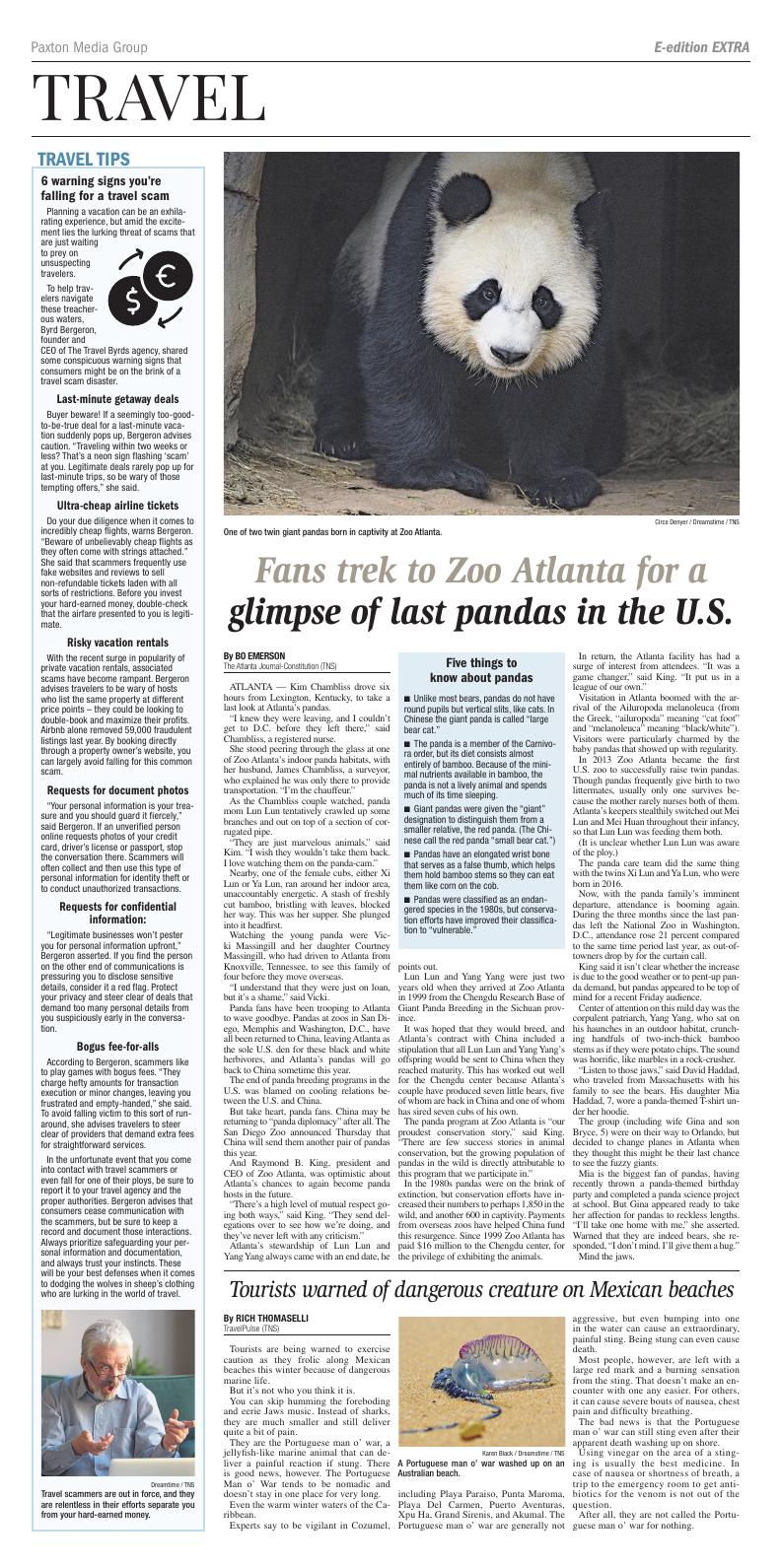The image depicts a newspaper's travel section, with various features and articles arranged in a structured format. In the top left corner, the words "Text and Media Group" are printed in small text. On the top right, the words "E-EDITION, E-EDITION, EXTRA" are prominently featured. Below this, the main headline bar showcases the word "TRAVEL" in large, bold black text.

The page is divided into three main sections:

1. **Left Section**: A blue column labeled "Travel Tips" runs from the top to the bottom of the page. The text within this column is too small to decipher. At the top right of this section, there's an image showing a coin with a dollar sign and another with a euro sign, with arrows indicating currency exchange. At the bottom of this column, there's an image of an older man with a shocked expression, sitting in front of a computer with his arms extended dramatically.

2. **Middle Section**: Dominated by an image of a panda bear looking directly at the camera. Below the image, an article headline reads: "Fans trek to Zoo Atlanta for a" in gray text, followed by "glimpse of last pandas in the U.S." in black text. The article appears to be divided into three columns. One of these columns is half-colored in blue, titled "Five Things to Know About Pandas," although the accompanying text is too small to read.

3. **Right Section**: At the bottom, there's a boxed warning with an image of a jellyfish on sand. The headline reads, "Tourists warned of dangerous creature on Mexican beaches," with article text surrounding the image.

This detailed composition captures the essence of a vibrant and informative travel section, filled with tips, intriguing articles, and vivid imagery.